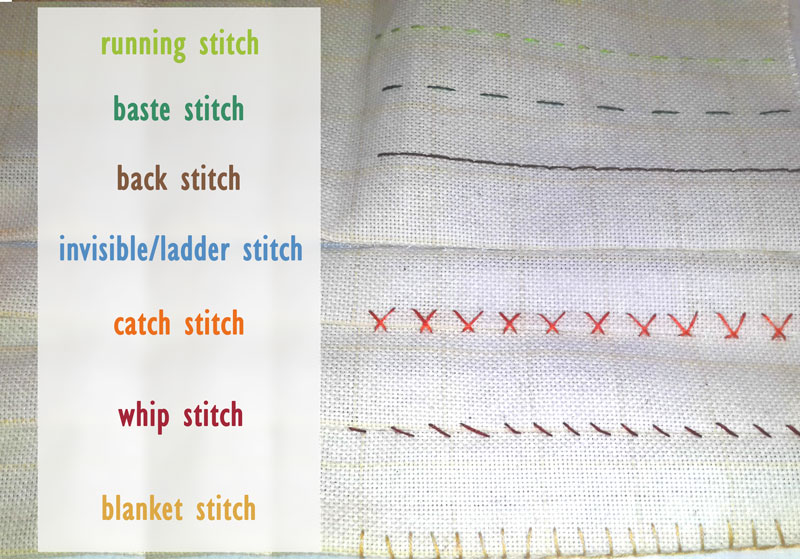The image showcases a brightly lit and clear photograph of a white fabric displaying various types of stitching. The fabric is divided into two sections: the left side features a tall, white rectangular legend with the names of seven different stitches, each written in a color that matches its corresponding stitch on the fabric. The list includes: 

1. Light green - Running stitch
2. Dark green - Baste stitch
3. Brown - Back stitch
4. Blue - Invisible/Ladder stitch
5. Orange - Catch stitch
6. Maroon - Whip stitch
7. Gold - Blanket stitch

On the right side of the fabric, the different stitching patterns are displayed, with each pattern executed in the same color as its label on the legend. The lines and shapes of the stitches vary, including green dotted lines, black dotted lines, straight lines, red X's, and yellow lines. The image is exceptionally detailed, capturing the distinct textures and colors of each stitch type, set against the white fabric backdrop.